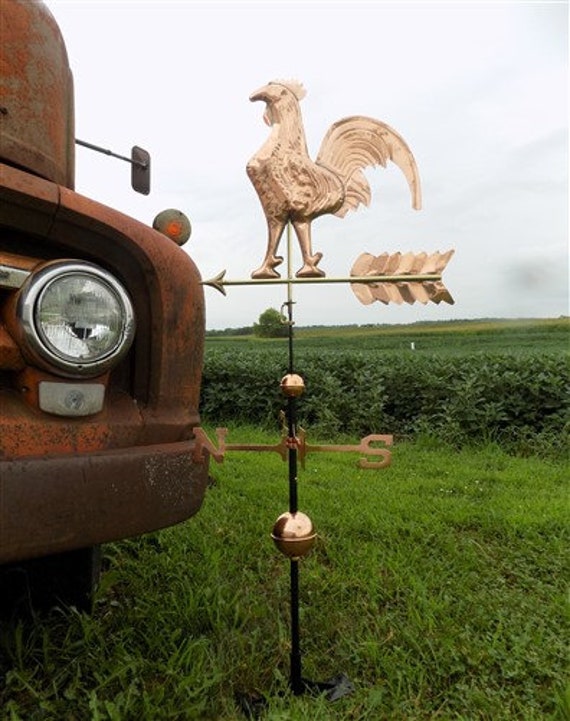The image portrays a weather vane in a vertical rectangular frame set against an outdoor backdrop. The weather vane, situated in the foreground, stands on a thin black metal pole rooted in ankle-high green grass. At the top of the pole is a golden rooster attached to a white horizontal bar with an arrow pointing to the left and gold feathers on the other side. Below the rooster, the black rod continues downward, punctuated by a gold ball, and further down, there's another gold ball. Between these balls, a horizontal softer gold rod indicates the cardinal directions with an 'N' for north on the left and an 'S' for south on the right. The weather vane is positioned near the front of a rusted-out, burnt-orange, and brown truck, where a shiny headlight and part of the side view mirror are visible. The background showcases a cloudy, light gray sky with patches of darker gray and an extensive field filled with tall green crops.